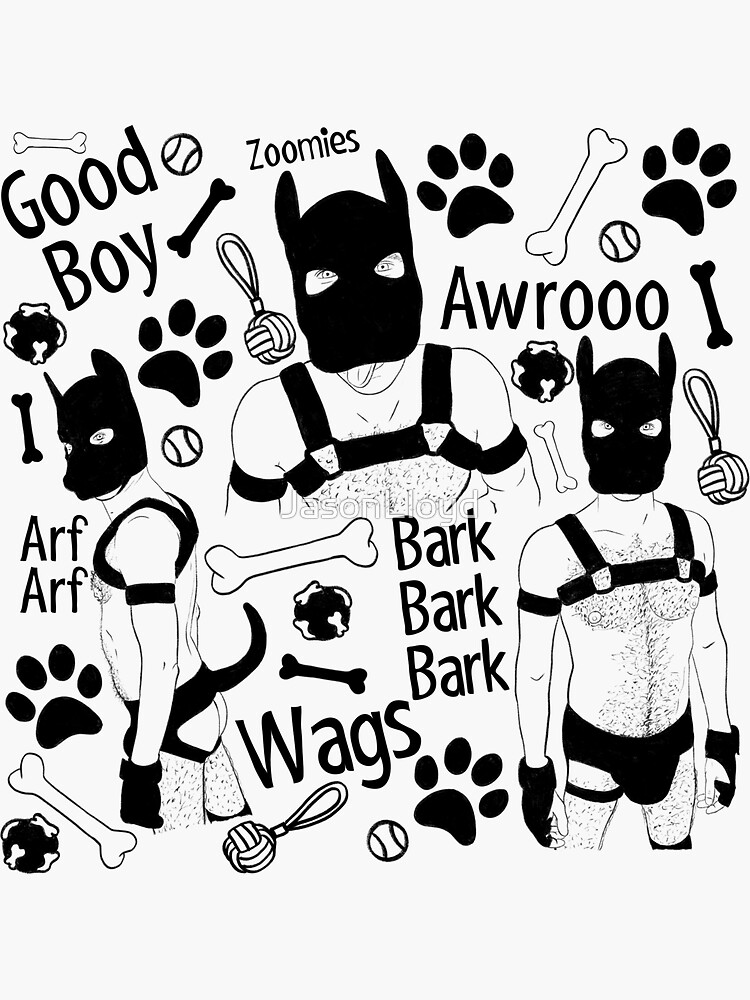This detailed black-and-white drawing depicts a man engaged in a fetish theme in which he pretends to be a dog. The artwork shows the same man in three different views: on the left, he is facing left but looking back at the viewer; in the top center, he is facing head-on, visible from the midsection up; and on the lower right, he is also facing the viewer. The man wears a dog hood that exposes only his eyes and features a tongue at the bottom, possibly part of the hood or his own if he has a long face. He is clad in bondage gear, including a harness, gloves, and undergarments with a tail at the rear, exposing his buttocks.

The image is peppered with various phrases in different fonts and sizes, such as "good boy," "zoomies," "aroOO," "arf arf," "bark bark bark," and "wags," all rendered in black text. There are also paw print designs, bones, and dog toys scattered throughout the composition, reinforcing the canine theme. The drawing is signed with a watermark that reads "Jason Lloyd," and the man is depicted looking at the viewer in each illustration, enhancing the engaging and somewhat provocative atmosphere of the artwork.